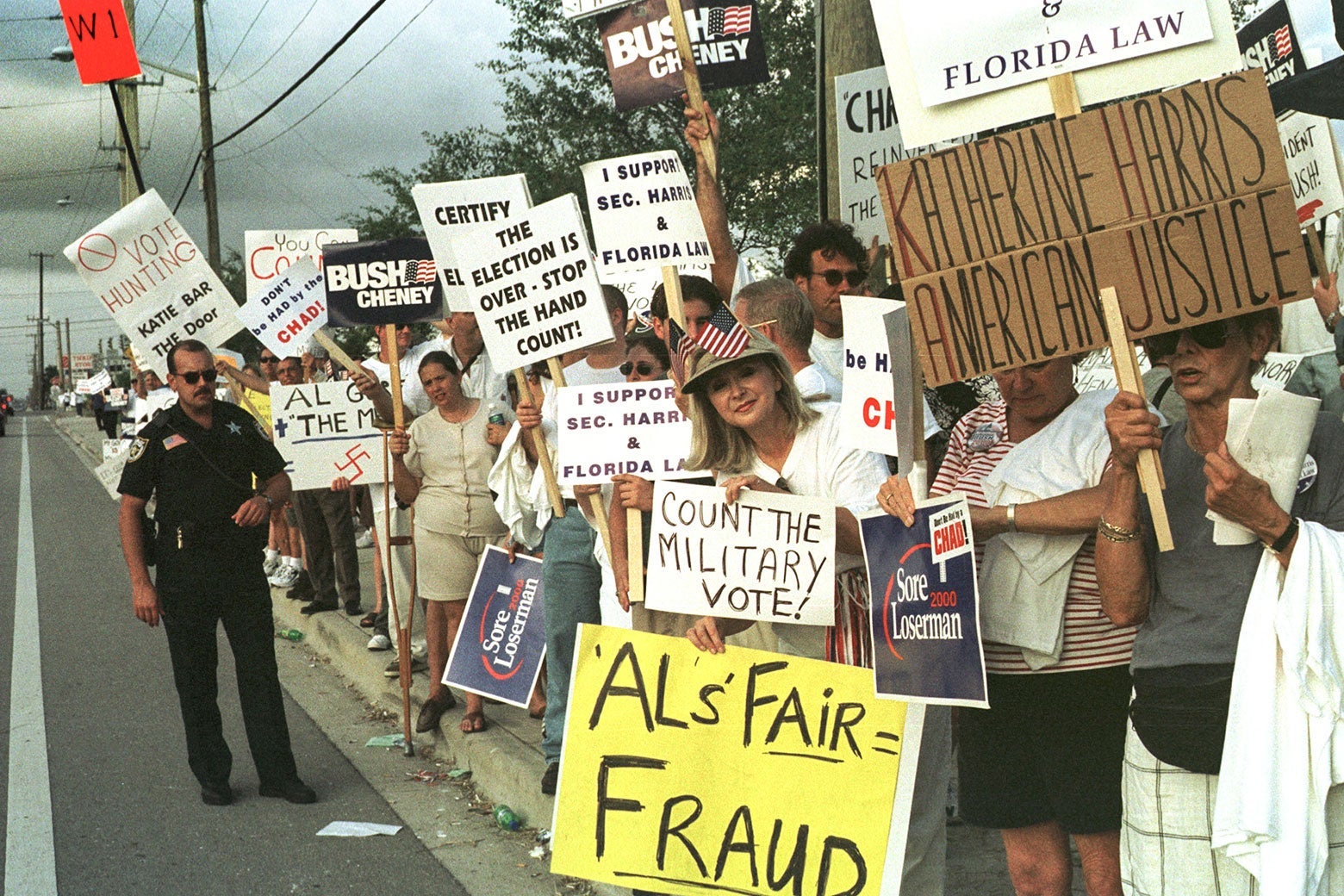This snapshot captures a cloudy day outside, showing a long line of protesters stretching down a sidewalk. The scene is dominated on the right side of the image by focused and large protesters, with a multitude of different types and races of people holding various signs. The signs feature different materials, ranging from cardboard to poster board, and include messages like "Bush-Cheney," "Katherine Harris, American Justice," and "Al's Fair Fraud."

In front of the picket line, a policeman stands by the curb, distinguishable in his sunglasses, short hair, black short-sleeved shirt, and long black pants. He faces the camera with his right arm by his side and his left arm bent at his waist, fingers pointing forward. The image also captures the details of the street's white line, a gray strip adjacent to it, and the trash littering the gray sidewalk.

The photograph hints at a political rally, given the nature of the signs and the era referenced by the "Bush-Cheney" sign. The protesters wear mostly white or tan shirts, with some donning hats. In the background, the scene includes a blue sky partially obscured by dark clouds, a tree line, and three power poles with hanging power lines. This detailed moment preserves the energy and diversity of a politically charged picket line.